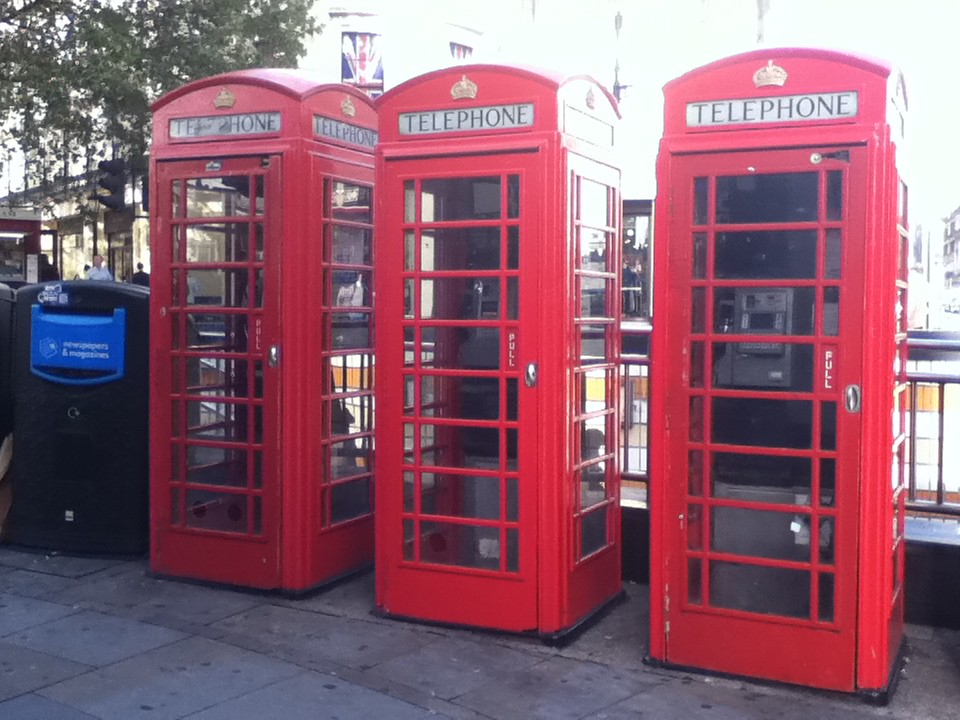This photograph captures a quintessential London scene featuring three iconic red telephone booths, lined up side by side. Each rectangular booth is adorned at the top with a gold crown and the word “TELEPHONE” boldly displayed in white capital letters against a black background. The clear windows allow a glimpse of the still-contained telephones, a rarity in modern times. A silver handle with a white "PULL" inscription graces each booth door. The backdrop reveals a bustling commercial area with white buildings, and a Union Jack flag in one of the windows. To the left, a black traffic light and a nearly indiscernible black box with blue and white markings are visible. Additionally, green tree branches and a metal railing suggest proximity to a street corner or possibly near a tube station. People can be spotted walking around, adding to the lively urban atmosphere.